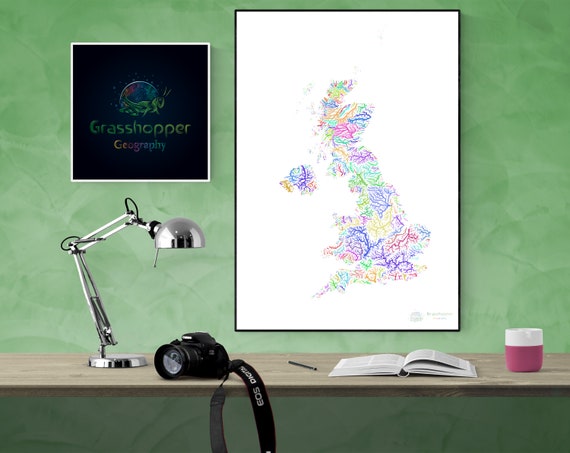The image features a neatly organized wooden desk set against green-painted walls. Positioned on the left side of the desk is a silver jointed lamp with articulating arms, allowing for directional lighting. Next to the lamp sits a sophisticated 35-millimeter camera with a black strap draped over the edge of the desk. An open workbook lies to the left, accompanied by a pen, further emphasizing the workspace ambiance.

Toward the right of the desk, a red and white coffee cup adds a splash of vibrant color. Above the desk area hangs an art piece in a black frame set against a white background. This piece showcases an abstract representation of the UK and Ireland, filled with a chaotic yet colorful array of pastels including purple, green, yellow, pink, and red. Next to this, another framed artwork rests on a dark background. This piece depicts an artistic grasshopper in green, blue, and pink, labeled "Grasshopper Company" in green lettering, enhancing the eclectic and creative atmosphere of the workspace.